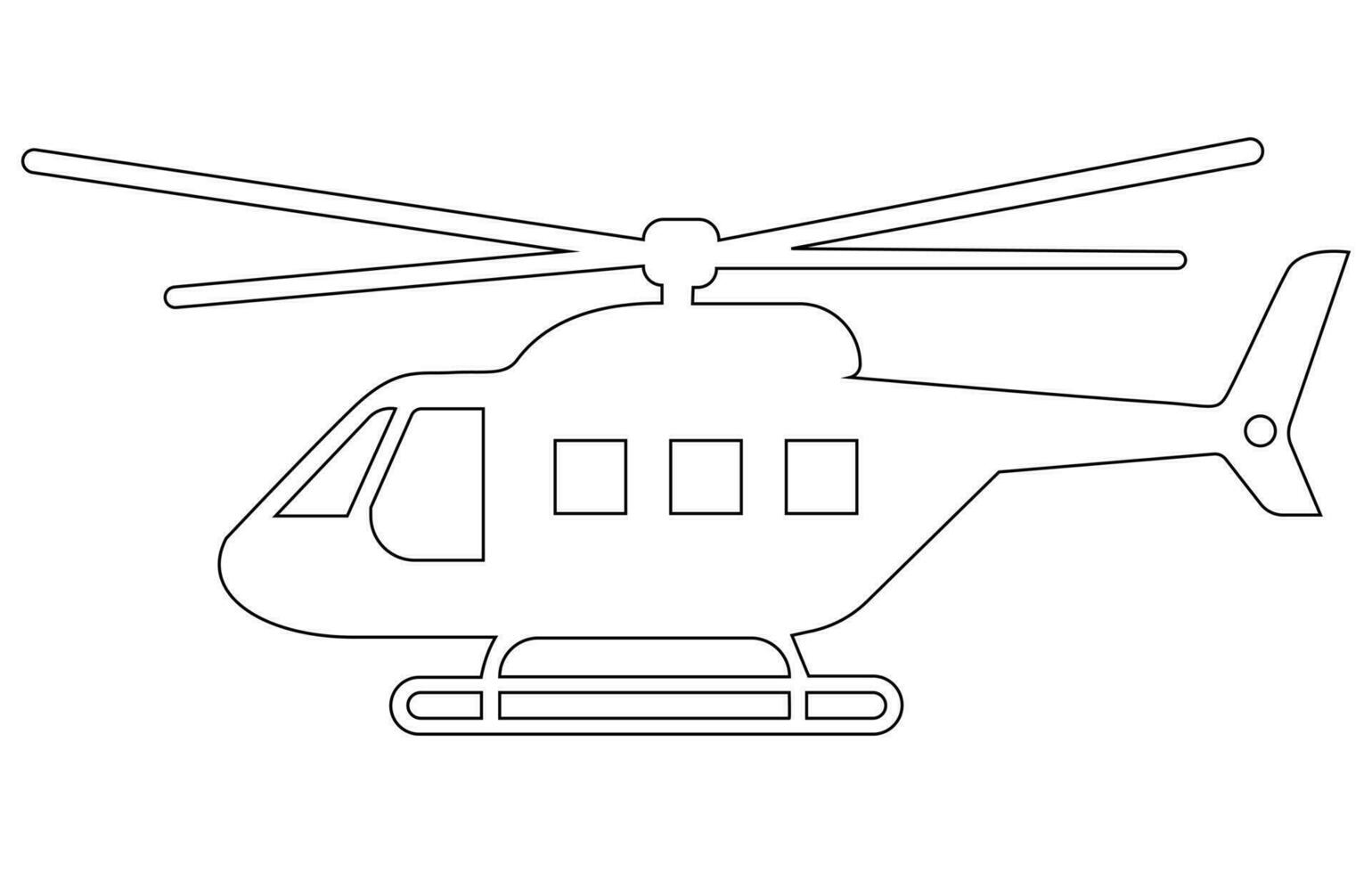This is a simple, black and white line drawing of a helicopter, rendered in black ink or a similar digital medium with precise, straight lines. The helicopter faces to the left, displaying four blades on top and a tail extending to the right. The body of the helicopter features a large door area, a windshield for the cockpit, and three smaller windows on the right side of the door. The landing apparatus consists of long, curved metal bars, suggesting it could potentially land on water. The helicopter appears to be suspended in a pure white, detail-free background, emphasizing its black outlines. No people are depicted in this straightforward but neatly executed drawing.